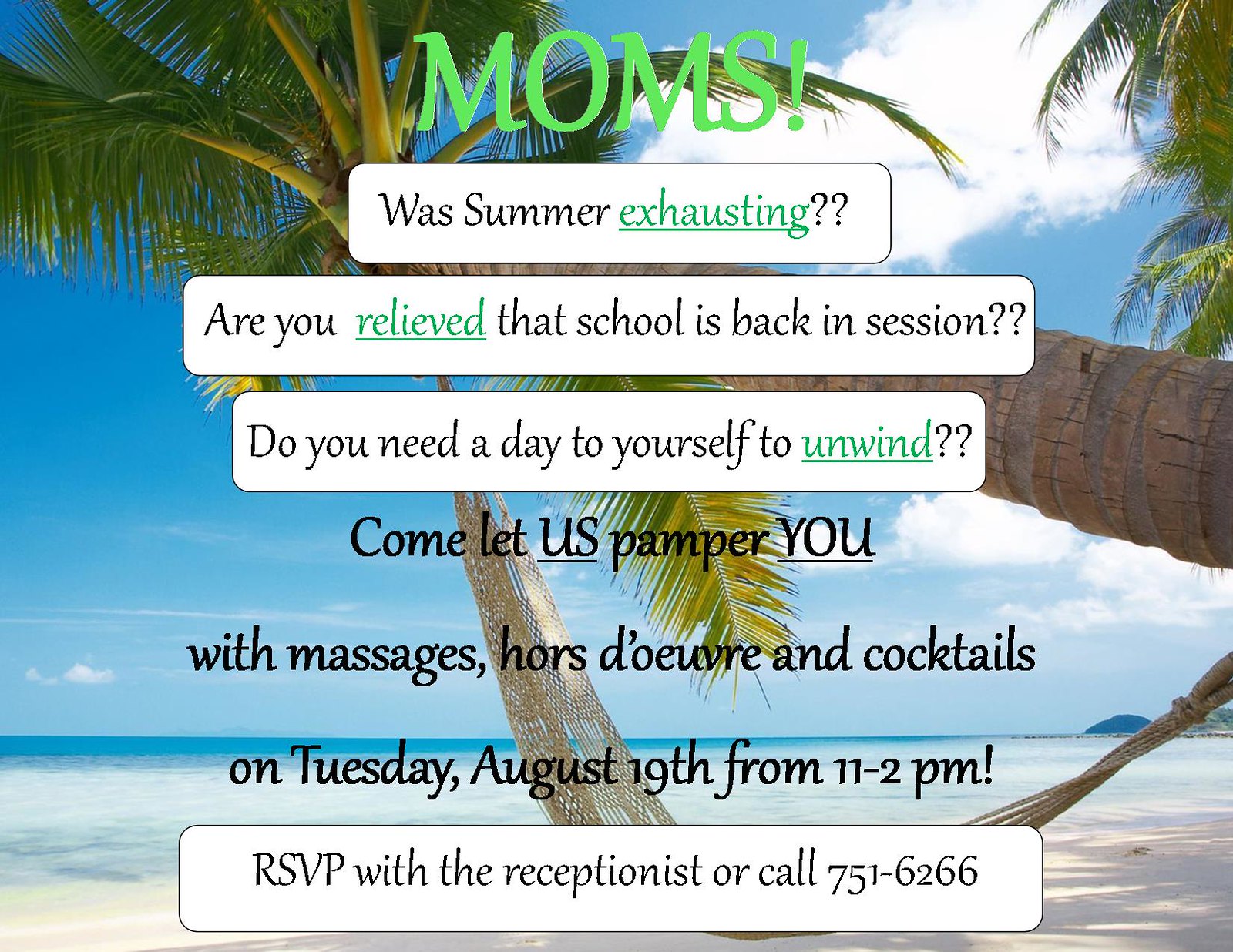The image is an advertisement set against a picturesque tropical beach background. A large palm tree arches gracefully over the scene, adorned with a beige hammock swaying gently. The pristine, white sand extends to the bright blue expanse of the ocean, where gentle waves meet the shore. Above, a stunning blue sky is dotted with fluffy white clouds, and there is a hint of a mountain visible in the distance.

Prominently displayed text, incorporating both green and black colors, addresses mothers directly: "Moms! Was summer exhausting? Are you relieved that school is back in session? Do you need a day to yourself to unwind? Come let us pamper you with massages, hors d'oeuvres, and cocktails." It specifies the event details: "On Tuesday, August 19th from 11 to 2pm, RSVP with the receptionist or call 751-6266." The words "exhausting," "relieved," and "unwind" are highlighted in green for emphasis.